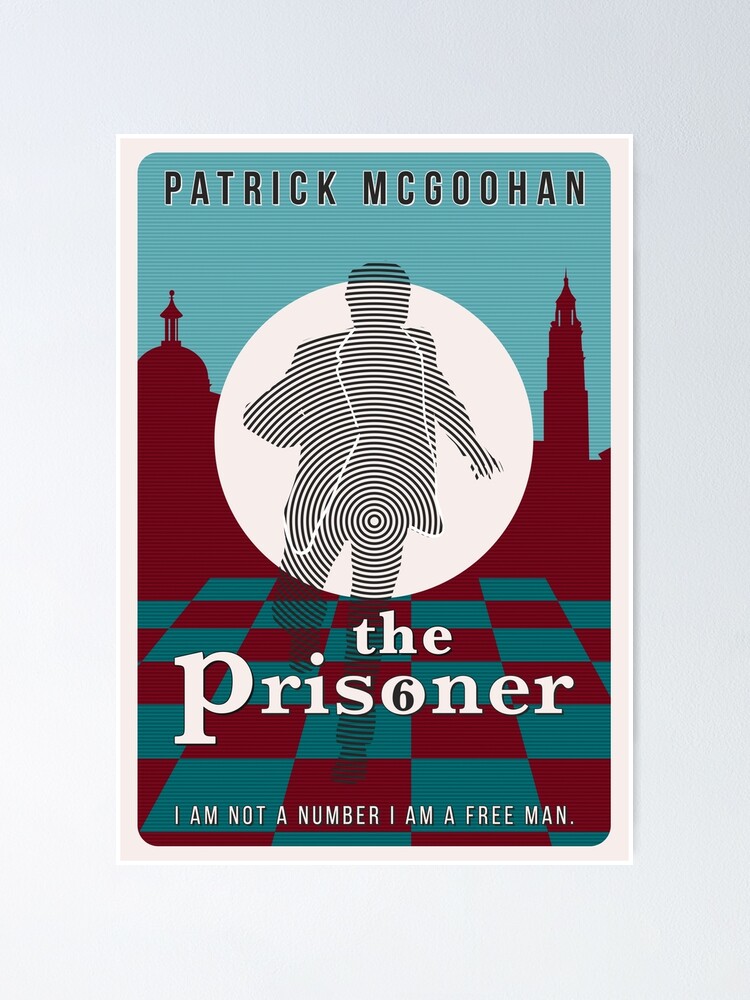The image is of a poster for the TV show "The Prisoner." The poster features detailed artwork on a cream-colored border set against a gray background. At the top of the poster, the name "PATRICK McGOOHAN" is prominently displayed in all uppercase black letters. The main section of the poster features a white rectangle with rounded edges, inside of which is a baby-blue rectangle — the background for the central artwork.

In the center of the baby-blue rectangle, there is a conspicuous white circle that contains the silhouette of a man in a suit, poised as if running. This figure stands atop a floor patterned in a red and light blue checkerboard style. Behind the figure, in solid red outlines, are various buildings including what appears to be a capitol building on the left and a church on the right, set against a light blue sky.

Towards the bottom of the poster, the title "The Prisoner" is written in white text. Within the word "Prisoner," the letter "O" contains a small number six. Below this, in smaller white text, reads the phrase: “I am not a number, I am a free man.” The poster is visually striking with its psychedelic zebra-like pattern silhouette, adding to its mysterious and captivating aesthetic.